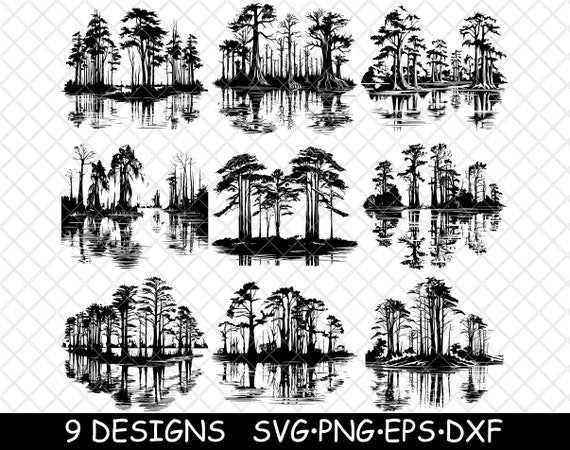This image features a set of nine black and white silhouette designs depicting various types of trees reflected in water. Each design showcases a different woodland environment, with variations in tree types—some resembling cypress trees common in swamps, perhaps like Louisiana's, and others appearing as tall pine trees. The scenes display a range of tree heights and densities, some with abundant foliage and others with sparse leaves. The designs are available in multiple formats, including SVG, PNG, EPS, and DXF, and are overlaid with a checkmark pattern to prevent copying. The caption “nine designs” in white text is positioned against a small black border at the bottom of the image, above a gray grid-patterned background.